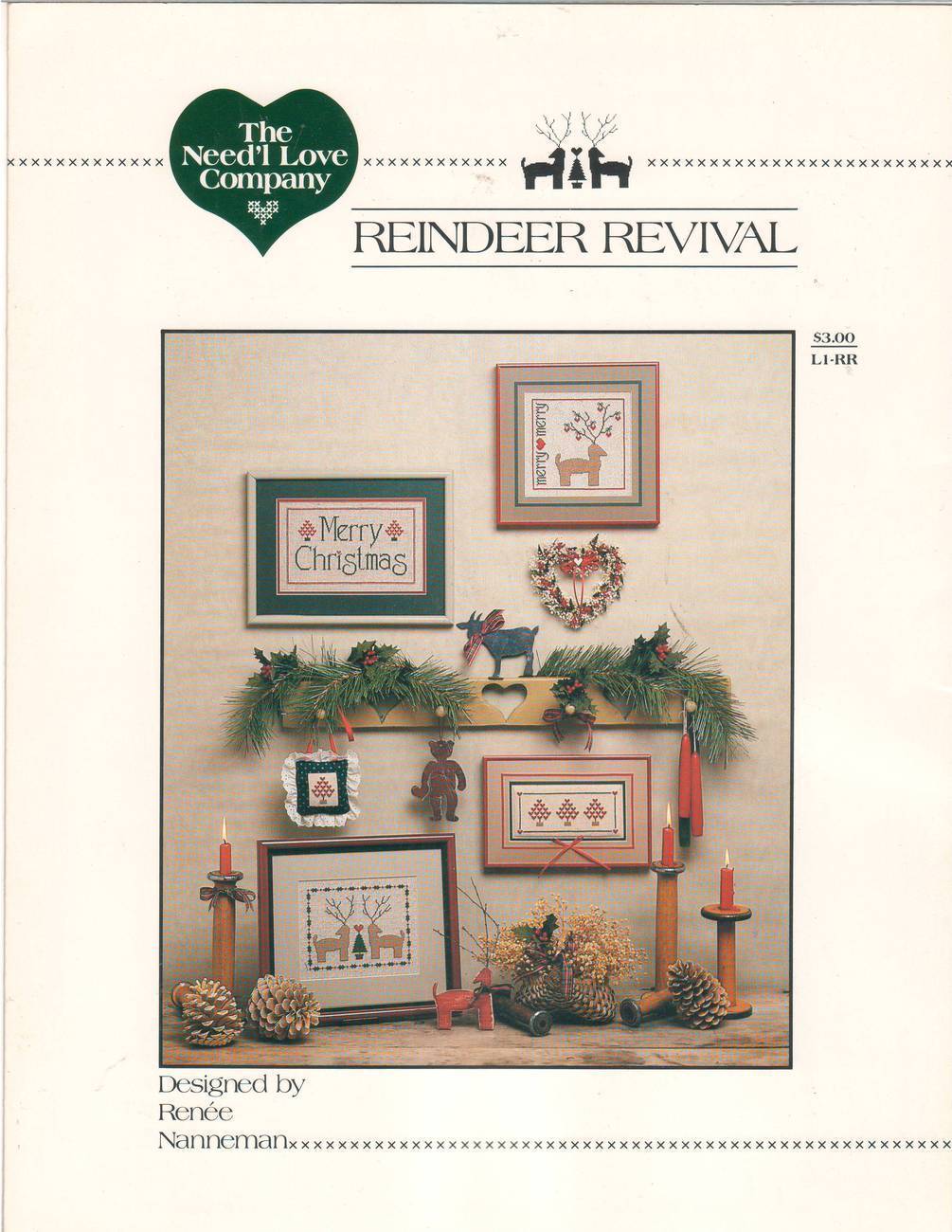This is a vertically-aligned rectangular advertisement page with a light beige background and a thin black border at the top. At the very top is a dark green heart containing the text "The Needle ('N-E-E-D apostrophe L') Love Company" in white letters centered within the heart. Beneath this heart is a dashed line made of X's. Immediately below this line, centered in all caps black letters, is the title "REINDEER REVIVAL," framed by horizontal black lines above and below. Above the title are two outlined reindeer images with antlers. 

The main section of the page features a rectangular image depicting a cozy home decor scene. The background shows a wall adorned with several pictures, including one saying "Merry Christmas" and another featuring a deer with antlers. On the ground are pine cones, and on a wooden shelf with a heart cut-out is Christmas holly and candles in wooden holders. The shelf also has a dark brown frame with another image of two deer facing each other. In the lower left corner, it says, "Designed by Renee Nanneman" in black text. The overall ambiance of the advertisement captures a very Christmassy and festive theme.